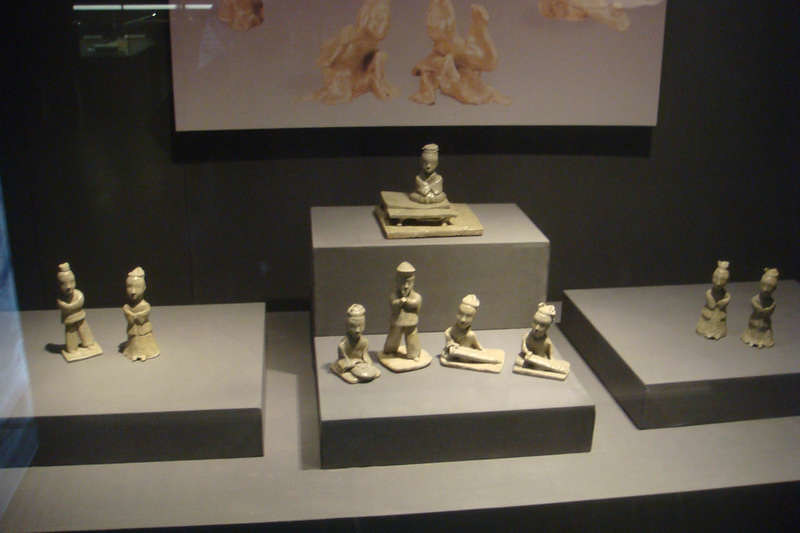This photo appears to be taken inside an Asian art or history museum, capturing a detailed exhibit of numerous small figurines displayed within a glass case. The exhibit features a variety of porcelain-looking statues, some resembling monks, arranged meticulously on four gray pedestals. The figurines, evocative of Asian cultural artifacts, are engaged in different postures and activities: from seated individuals with crossed legs or folded arms to standing figures, including women with hands together and men with arms folded. Adding depth and context, a partially visible painting or photograph of similar Asian-style figures hangs above the exhibit, reflecting the overall aesthetic theme. The reflection off the glass casing further confirms this as a carefully curated museum display.